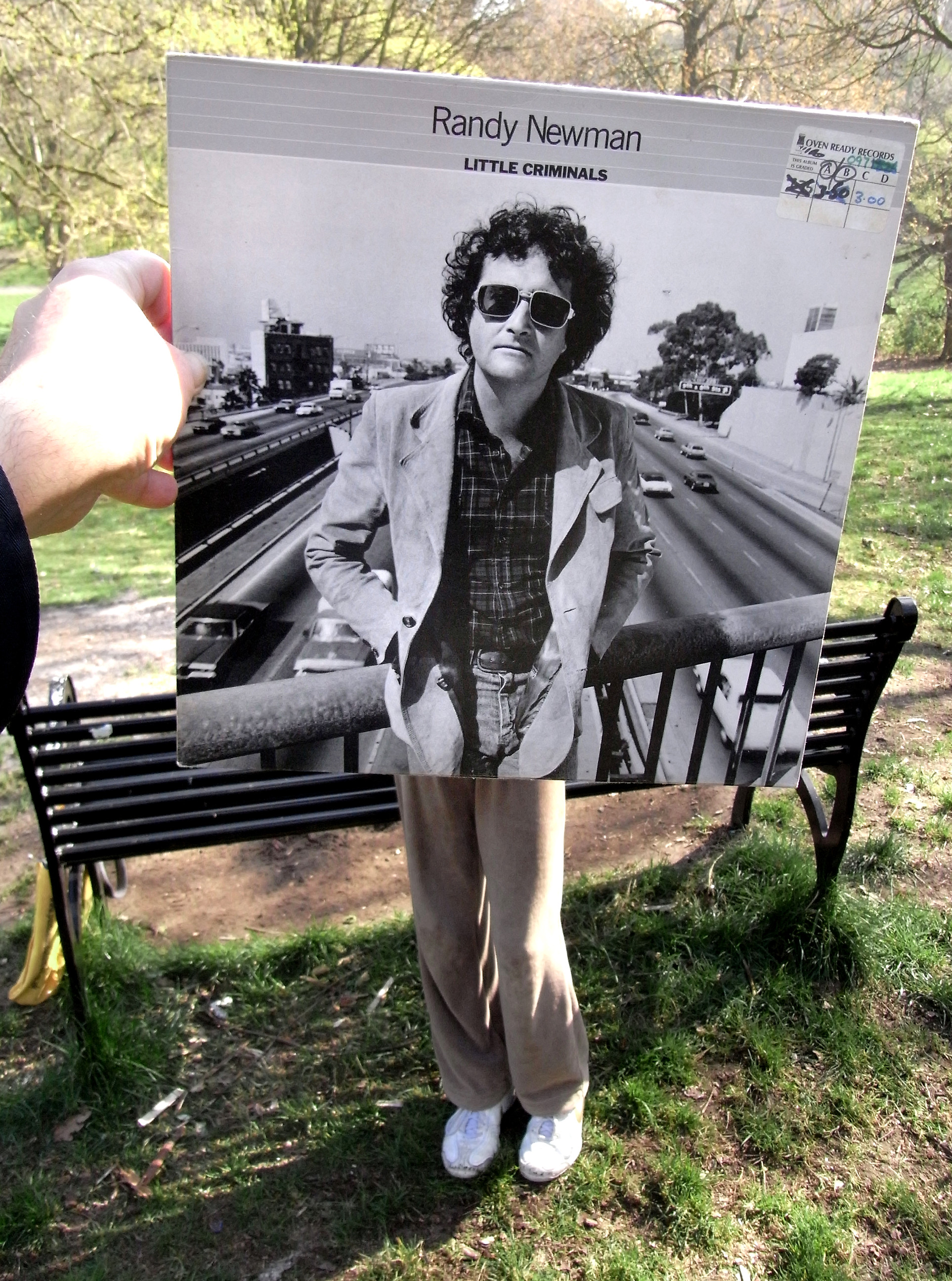The image depicts a person standing in a park, holding up a vinyl record cover in front of them. The album is "Little Criminals" by Randy Newman, featuring a black and white photo of Newman with curly brown hair, wearing sunglasses, a jacket, and a collared shirt. The cover shows him leaning over a railing, overlooking a busy highway with cars and a distant tree visible. Intriguingly, the person holding the album has positioned it perfectly, so that the legs of another individual wearing tan pants and white shoes appear seamlessly integrated as Newman's legs. This clever alignment creates a humorous and visually striking composite image, with the park's green grass, trees, and a bench visible in the background, all set in the daytime.